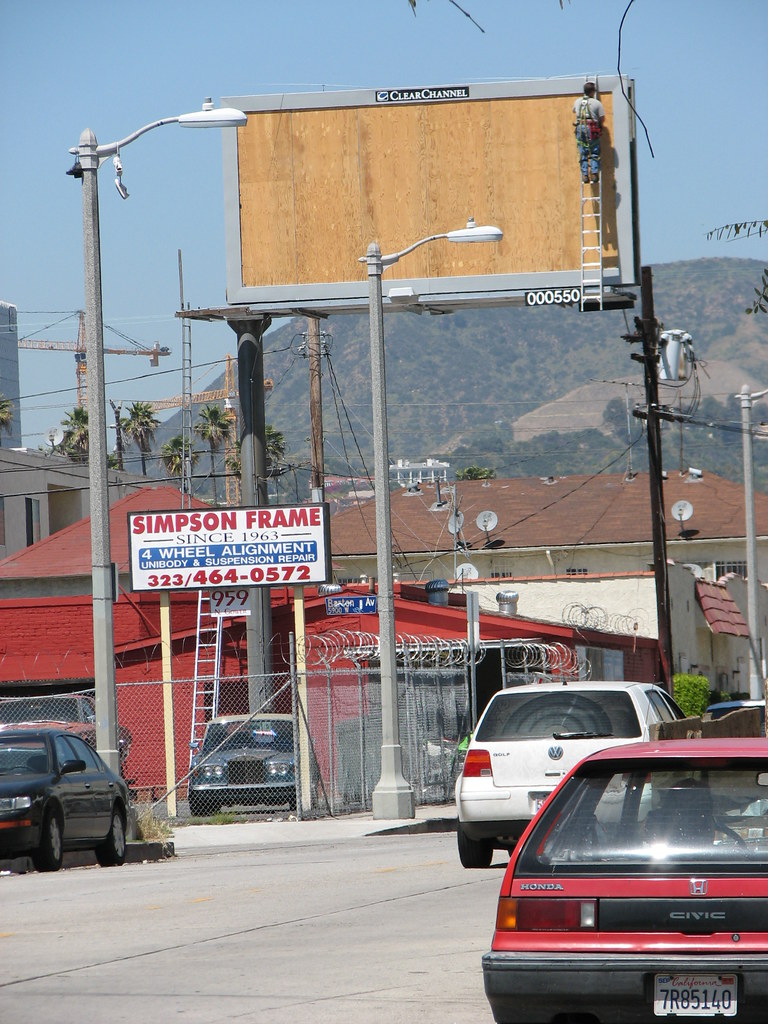This detailed photograph captures a bustling downtown area with a clear blue sky and a hazy mountainous backdrop. Dominating the foreground is a city street where a red Honda Civic with a California license plate and a white Volkswagen Golf are visible, the latter driving down the road. A black car is parked on the opposite side of the street. A small, one-story red building is prominently featured, fortified by a chain-link fence topped with barbed wire. This business, identified by a sign reading "Simpson Frame since 1963," offers four-wheel alignment, unibody, and suspension repair services, with the phone number 323-464-0572 listed below.

Within the fenced area, a luxurious car, possibly a Rolls Royce or Bentley, can be seen. Above this building, an imposing billboard looms, with a "Clear Channel" label at the top. The billboard is in the midst of refurbishment, evidenced by the presence of plywood and a man precariously perched on a seemingly floating ladder, working on the structure. A streetlight and the intricate details of a silver ladder inside the fenced area add to the bustling, industrious atmosphere of the scene.